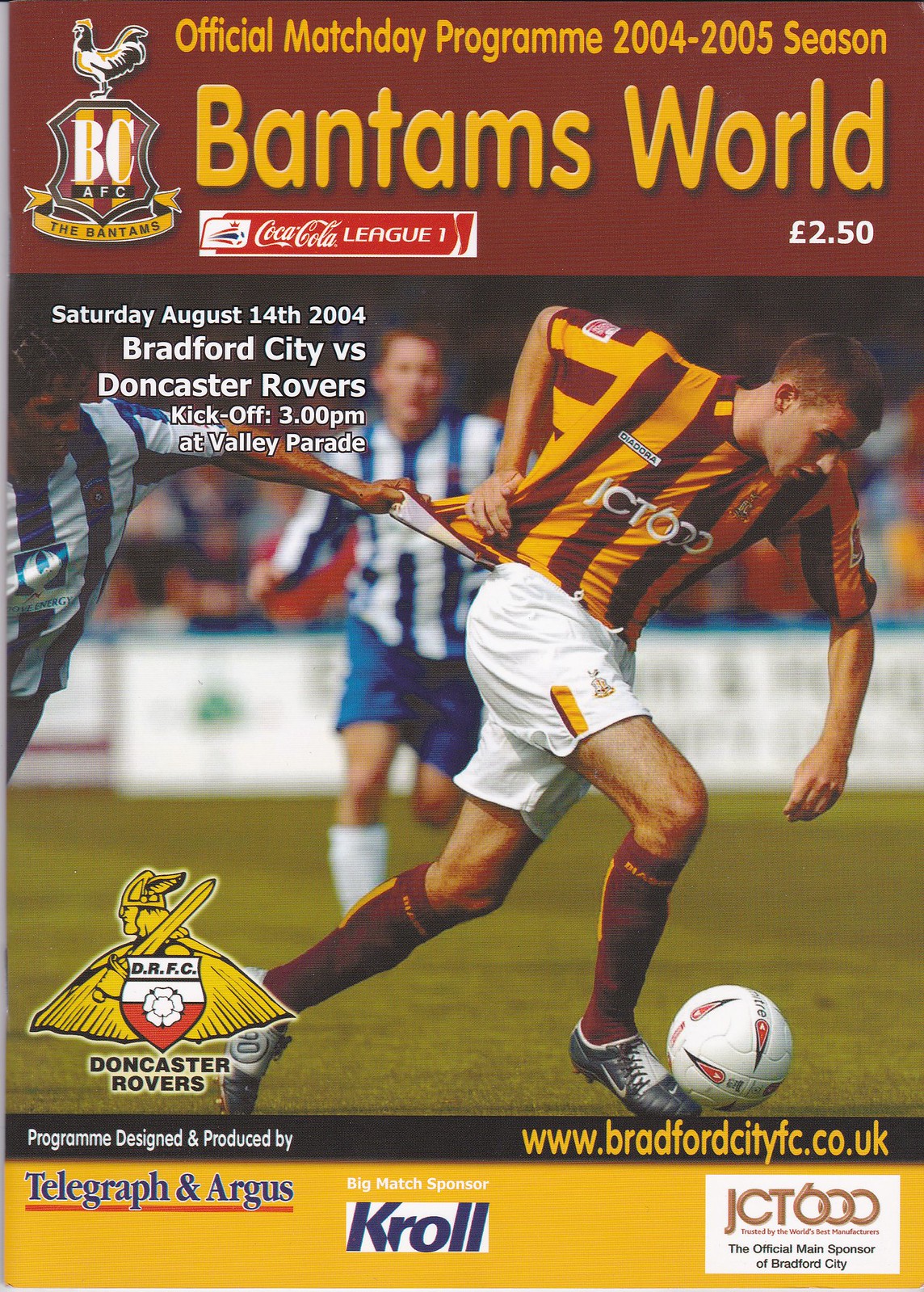The image features the front cover of an official match day program for the 2004-2005 season, titled "Bantams World." At the very top of the cover is a red rectangle with yellow text reading, "Official Match Day Program 2004-2005 Season." Directly below, the text "Bantams World" is prominently displayed, accompanied by the Coca-Cola League One branding. On the top right, the price is marked as £2.50. In the middle left section, the date "Saturday, August 14, 2004" is given in white text, with the match details "Bradford City vs. Doncaster Rovers" below it. The kickoff time, "3 p.m." and location, "At Valley Parade," follow beneath.

The central image on the cover captures an intense soccer moment: a Bradford City player wearing a yellow and burgundy vertically striped jersey with "JCT 600" on the front, paired with white shorts, is being pulled on by a Doncaster Rovers player. The Doncaster player is dressed in a red and white vertically striped jersey with "Dove Energy," featuring a picture of a dove, and white shorts. Another Doncaster player is seen approaching in the background. The backdrop shows the soccer field in action.

At the bottom, the cover includes text promoting www.bradfordcityfc.co.uk and mentions sponsors such as "Telegraph and Argus," "Kroll," and "JCT 600," noted as the "trusted by the world's best manufacturers" and the "official main sponsor of Bradford City." The Doncaster Rovers emblem, depicting a viking and a soldier, is also present, contributing to the overall design and informational content of the program cover.